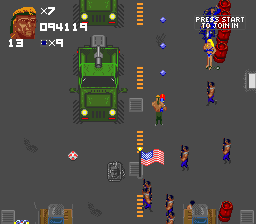A nostalgic snapshot from a retro video game, likely from the late 80s to early 90s, characterized by its pixelated graphics and vibrant colors. The scene features eight characters, with one prominently positioned in the foreground, armed with a gun-like object that shoots three blue, circular bullets into the air. Adjacent to this character, a convoy of green jeeps is driving downward along a grey road marked with yellow dashed stripes, adding to the action-packed dynamics of the image.